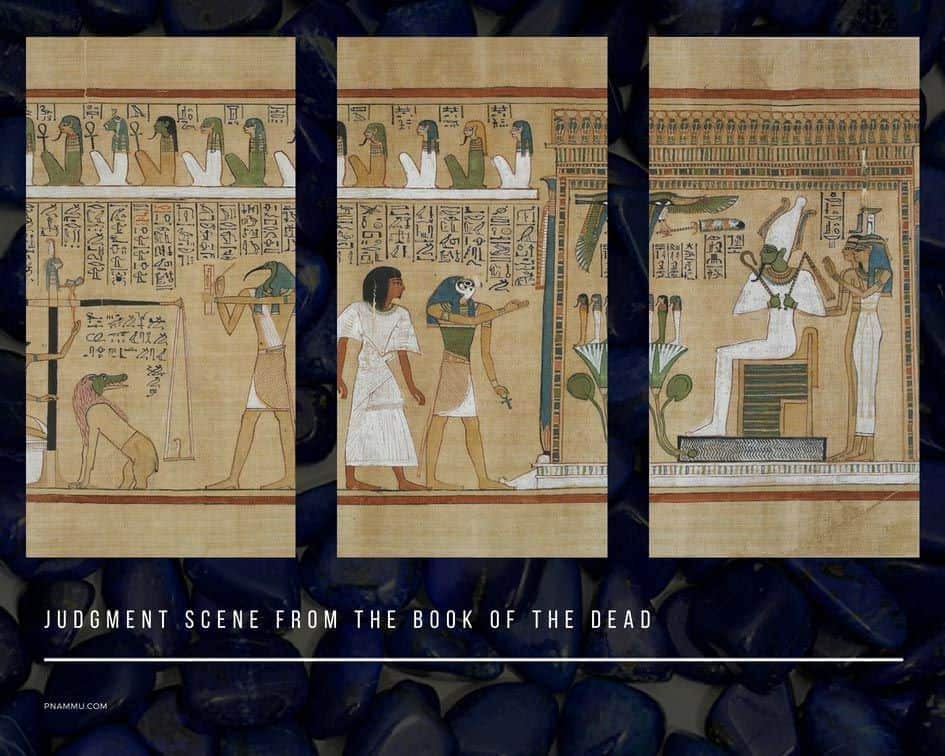The image presents an intricate scene from the Book of the Dead, characterized by an Egyptian style of artistry. The primary backdrop features a textured display resembling faded blue rocks or shiny blue pebbles. Central to the imagery, various figures stand arranged in a notable pattern, their hues ranging from beige and brown to green and white, complemented by the overarching beige background of the artwork.

Prominently, there's a depiction of a person with dark skin and dark hair, adorned in a white dress, being guided by a figure with a human body and a bird's head towards a throne. The figure on the throne, also garbed in white with a matching hat, is flanked by two women standing behind them. Additionally, a peculiar figure, an amalgamation of a dog and an alligator’s face, and another humanoid form with the head of a bird can be seen.

Inscriptions at the base of the image read "Judgment Scene from the Book of the Dead" in white text, accompanied by a horizontal white underline. A URL—p-n-a-m-m-u dot com—is located in the bottom left corner. The picture is both vibrant and nuanced, steeped in the rich aesthetics and symbolism of ancient Egyptian lore.